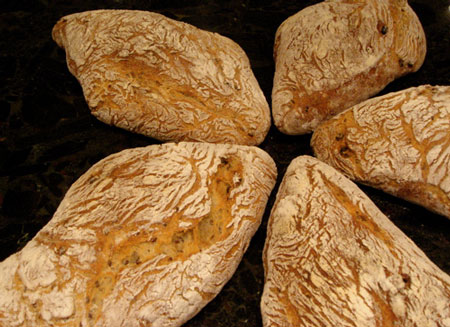In this square image, set against a solid black background, there are five brown objects arranged in a circular formation. These oblong, grooved items, reminiscent of rough, textured baked potatoes or perhaps unusual rocks, narrow towards their rounded ends which all point to the center, creating a focal black area. The largest object resides in the lower left corner, with others positioned in the upper left, upper right, coming in from the right side, and the lower right. Some of them extend beyond the visible frame. The light to medium brown objects exhibit a rough, crusted appearance, and traces of powdery residue hint at a baked or earthy origin. Despite their mysterious nature, they seem deliberately positioned, forming a unique and cohesive arrangement.